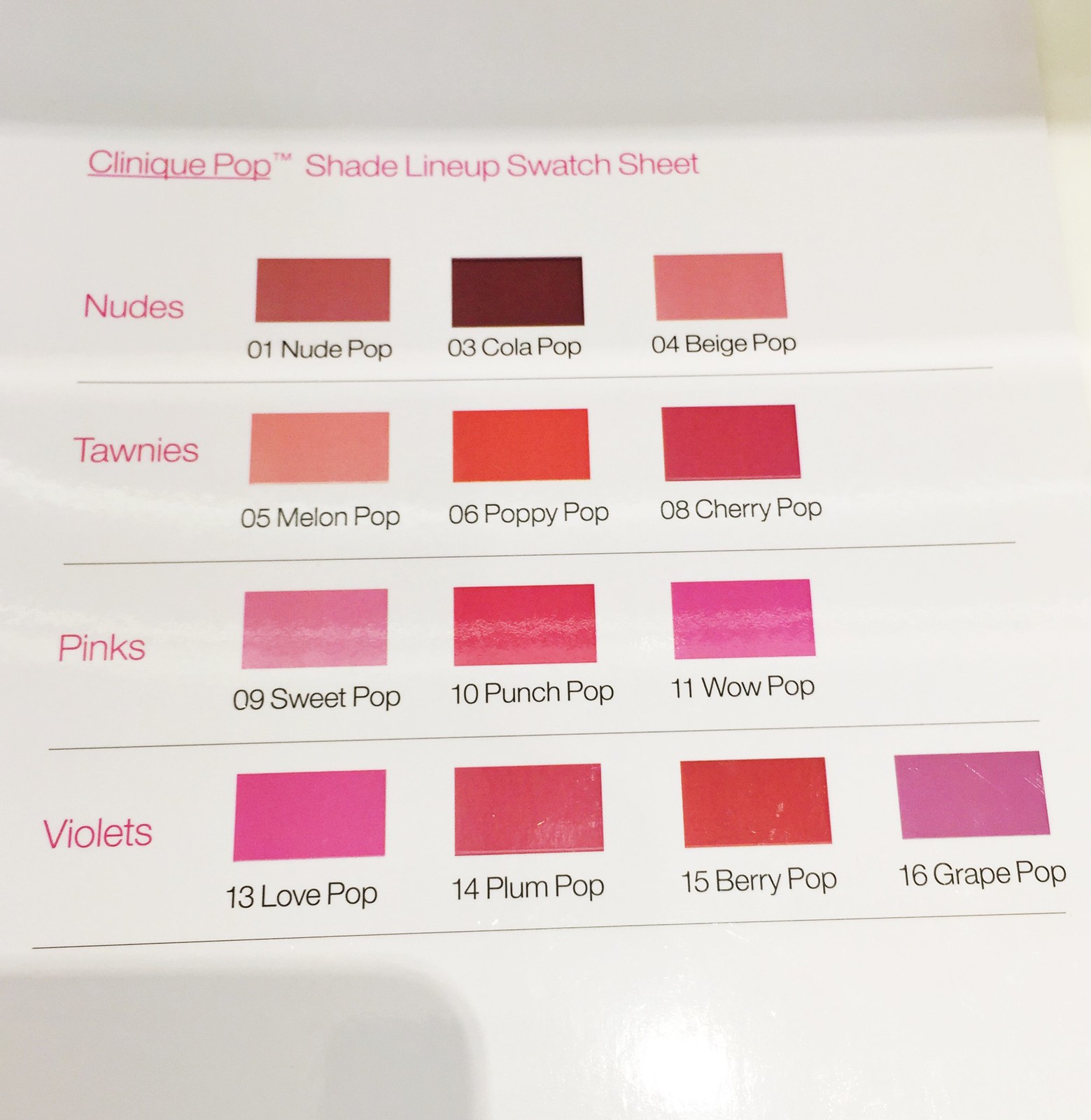The image displays the Clinique Pop Shade Line-Up Swatch Sheet against a white background. The top features pink text reading "Clinique Pop™ Shade Lineup Swatch Sheet." There are four rows categorizing the shades into Nudes, Tawnies, Pinks, and Violets, each category labeled at the beginning of the row in pink text. The nudes include 01 Nude Pop, 03 Cola Pop, and 04 Beige Pop. The tawnies cover 05 Melon Pop, 06 Poppy Pop, and 08 Cherry Pop. The pinks consist of 09 Sweet Pop, 10 Punch Pop, and 11 Wow Pop. Lastly, the violets are 13 Love Pop, 14 Plum Pop, 15 Berry Pop, and 16 Grape Pop. Each shade is represented by a colored rectangle with its corresponding name and number written in black text below it, showcasing an array of pink and red hues.